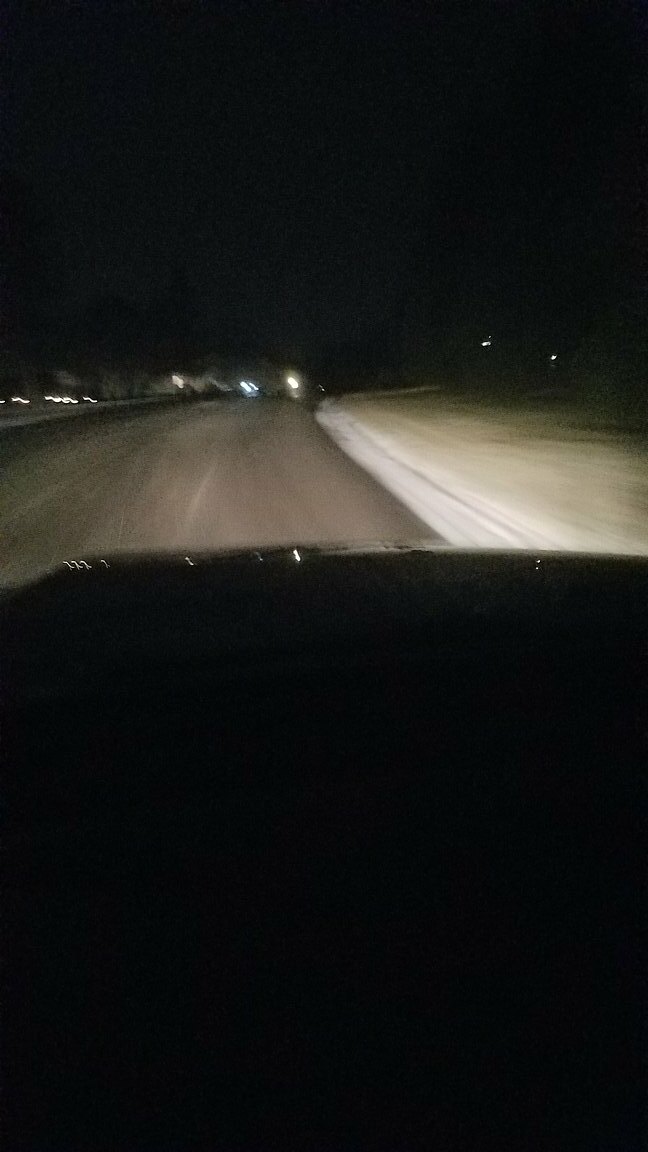A blurred nighttime photograph captured from inside a moving vehicle on a highway. The bottom portion of the image appears completely black, possibly indicating the interior of the car with a slight glimpse of the car's dashboard. The road ahead is a gray blur, emphasizing the motion of the vehicle, with patches of snow visible along the right-hand side. The left side of the image features scattered lights, likely from distant vehicles or roadside fixtures, accompanied by more snow. The top third of the image is entirely dark, suggesting it’s nighttime. Faint silhouettes of trees are visible in the upper background, contributing to the overall dimly-lit, wintry atmosphere of the scene.